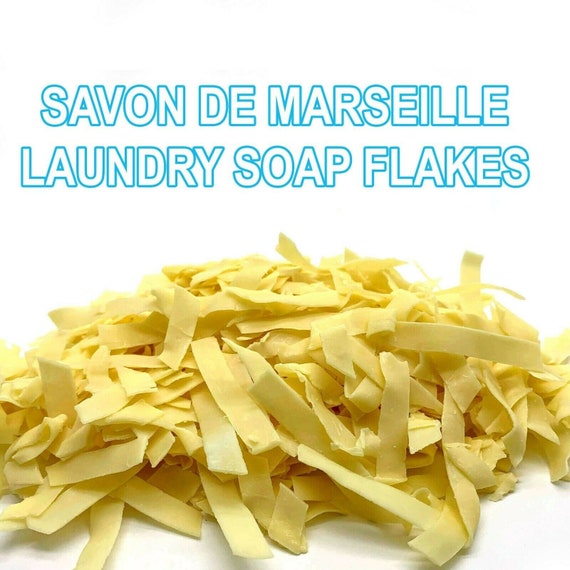The image portrays a product packaging with text in both English and another language, possibly Spanish or French. The top of the package has bold, capital letters with a blue outline and a white center that read "Savon de Marseille." Below this, it says "Laundry Soap Flakes." The soap flakes themselves are depicted in the lower half of the image, appearing as a pile of long, rectangular yellow chips. These chips resemble something akin to salad toppings or grated cheese. The backdrop of the image is a clean, white background that highlights the contrast and detail of the soap flakes, giving them a striking and clear presentation.